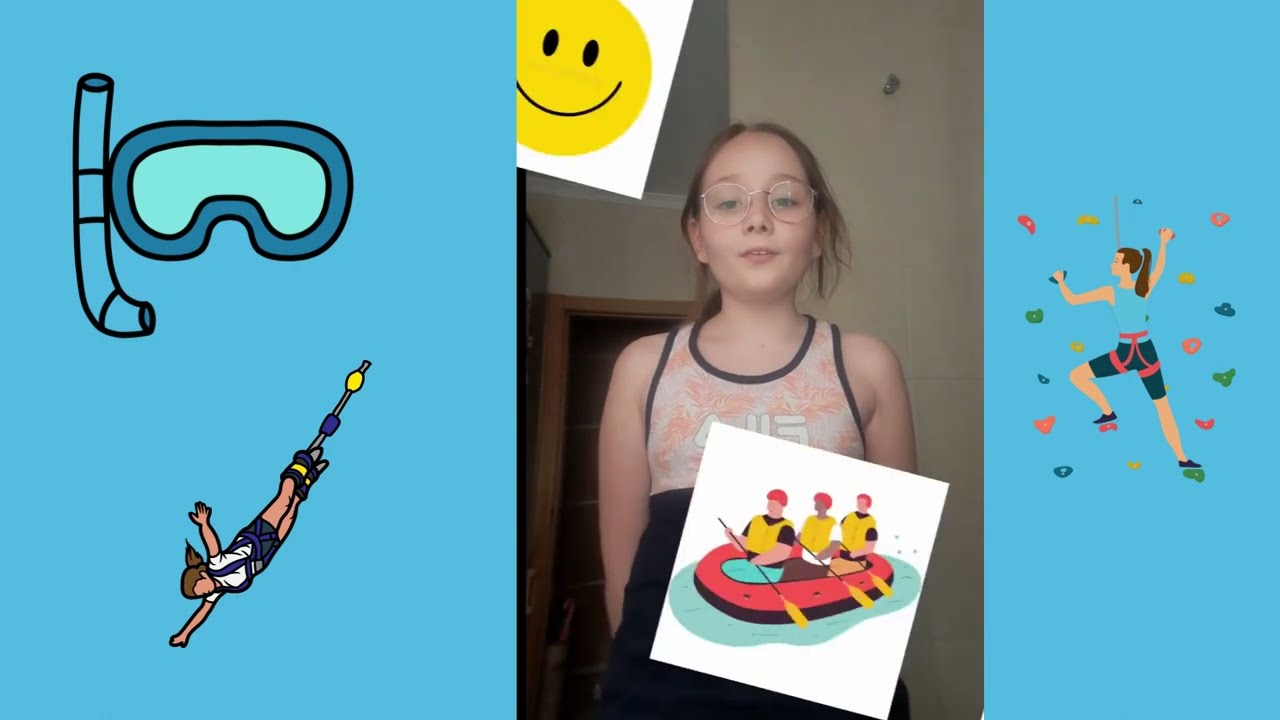The image is a color photograph in portrait orientation, inset into a blue background with various illustrations. The centerpiece is a cell phone photo of a young girl, about 9-10 years old, standing in a hallway at home. She has light skin, brown hair pulled back, and wears clear eyeglass frames along with a sleeveless dress featuring an orange design on top and a black bottom. She is smiling slightly with her mouth slightly open. 

Above her, to the left, is an angled yellow smiley face emoji. Below her is an illustration of three people in a red raft with gold oars. To the right in a blue section is a cartoon drawing of a woman climbing a rock wall, equipped with a harness, ponytail, blue shirt, and black shorts. On the left, also set against a blue background, is a diver's mask and snorkel illustration above another image of a woman bungee jumping with her arms outstretched. These surrounding images likely represent her various interests, combining elements of both illustration and realistic photography.